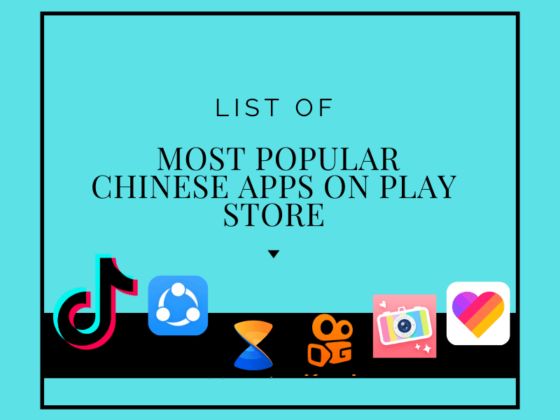This is an infographic featuring a prominent, central black-bordered box set against a blue background. Within the box, large, bold black letters announce "List of Most Popular Chinese Apps on Play Store," with the text centered for emphasis. Directly below, a downward-pointing arrow leads the viewer's eye to a horizontal row of social media app icons at the bottom. The icons include TikTok, two unidentified photo apps, one with a heart symbol, and a blue square app adorned with white circular dots. This infographic serves as an attention-grabbing headline photo or a social media post highlighting the most popular Chinese apps available on the Play Store.